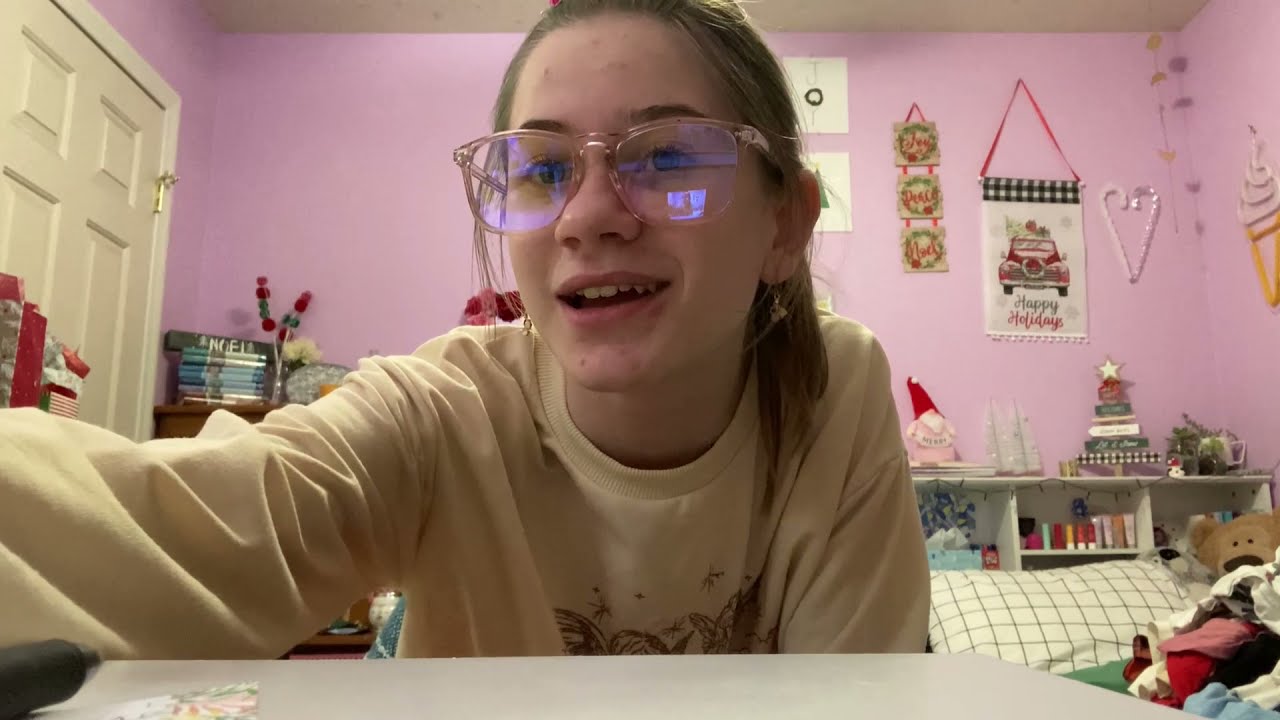A young teenage girl, possibly 13 or 14 years old, is sitting at her desk in her pink-themed bedroom, recording a video with a computer in front of her. She has light brown or blond hair pulled back into a ponytail and is wearing prescription glasses with soft pink, transparent frames. She is dressed in a cream-colored, long-sleeved sweatshirt and adorned with dangly earrings. The reflection of her computer screen is visible on her glasses, indicating she might be on a video call or recording content for YouTube or TikTok. She is smiling and appears to be engaging with her audience. The walls behind her are decorated for the holidays, featuring a "Happy Holidays" banner, a little wooden Christmas tree, and a Santa Claus figurine. Her bed, which has a headboard with at least three distinct sections, is home to several stuffed animals, including a large teddy bear and possibly a pile of clothes. The room is embellished with girly artwork and cute toys, creating a cozy and festive atmosphere.